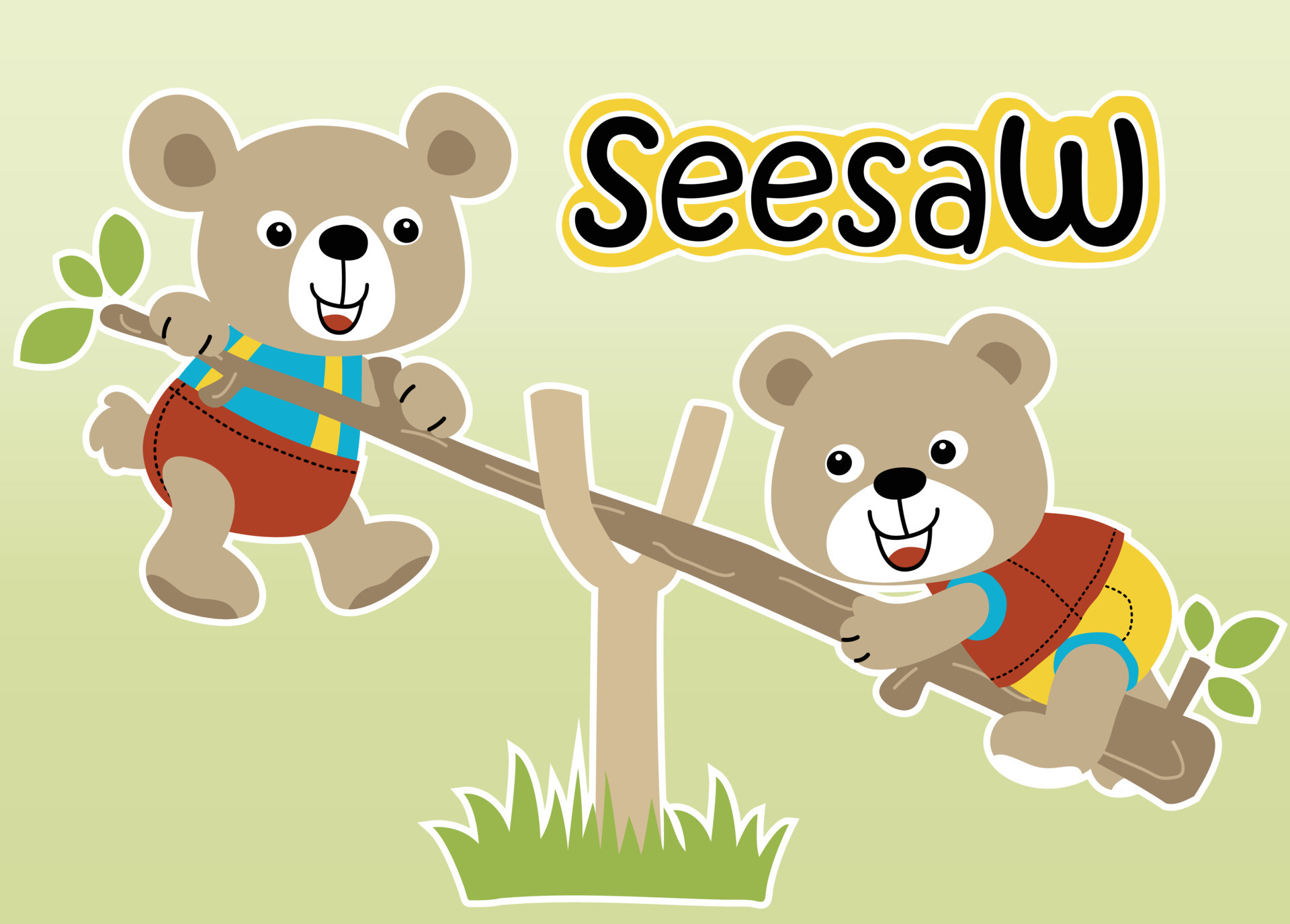In this charming children's illustration, two light brown bear cubs are captured in a moment of pure joy as they play on a makeshift seesaw crafted from a tree branch. The seesaw, composed of a long branch balanced on a U-shaped branch still adorned with a few leaves, serves as their playful pivot. The word "seesaw" is prominently displayed in black lettering with a yellow highlight at the top right corner of the image.

These endearing bear cubs are dressed in colorful attire, adding to the playful atmosphere. The bear on the right, positioned nearer to the ground and ready to push off, is wearing a red shirt with blue collar and shoulder cuffs paired with yellow pants featuring blue leggings. The bear on the left, soaring upwards, is clad in a blue shirt, red pants, and yellow overall straps. Both bears have wide, open smiles as they gaze at each other, their joy and laughter palpable. The background is a soft light green, enhancing the whimsical, joyful scene.